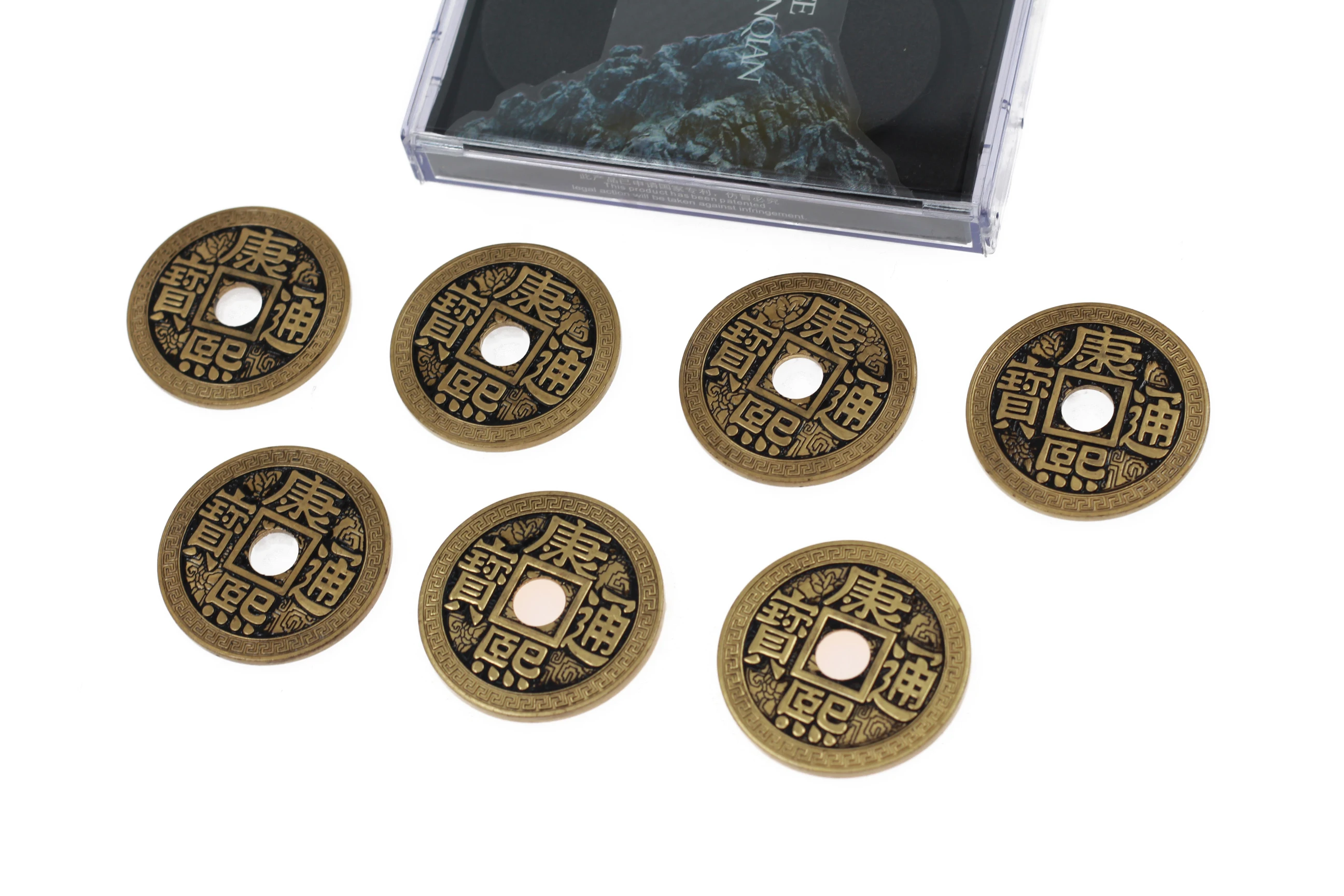This is a detailed photograph showcasing a set of seven traditional Chinese copper coins, reputed for bringing good luck or fortune. The brass-colored coins, imbued with Asian characters and symbols, are ornately designed with raised engravings and feature a circular hole in the center. These coins are arranged in two rows—four in the top row and three in the bottom row—set against a transparent background. Each coin has black shading, which appears to vary slightly in intensity, particularly around the top four and the bottom left coin. A partial view of a plastic clamshell box, perhaps the original container for the coins, is visible at the top of the image. The box displays a cut-off label showing the letters "N-O-I-A-N" and part of an "E," along with an image resembling rocks or a mountain. Additionally, there is an opaque rectangle and what could be interpreted as a digital screen body behind the coins, offering an intriguing backdrop that complements the antique quality of these auspicious coins.